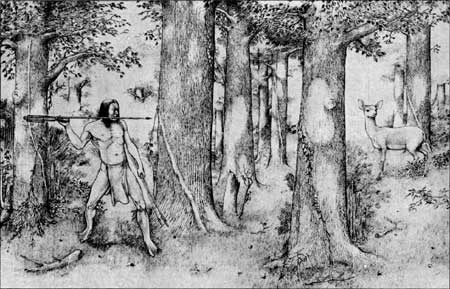The black-and-white photograph captures a dense woodland scene with several thick-trunked deciduous trees and scattered bushes. In the foreground on the left side, there is a barefoot Native American man with long hair, dressed in a loincloth. He stands with his legs apart, holding a spear-like weapon in his right arm, which is bent at the elbow, resting the spear behind his shoulders. His body faces slightly towards the viewer, while his head is turned to the right. On the right side of the image, a deer stands in profile among the trees, also facing left but turning its head to look towards the viewer. The scene includes a forest floor littered with grass and sticks, and the photo's landscape orientation gives a wide view of the forested area. The man and the deer create a dynamic tension as if in a hunting moment.